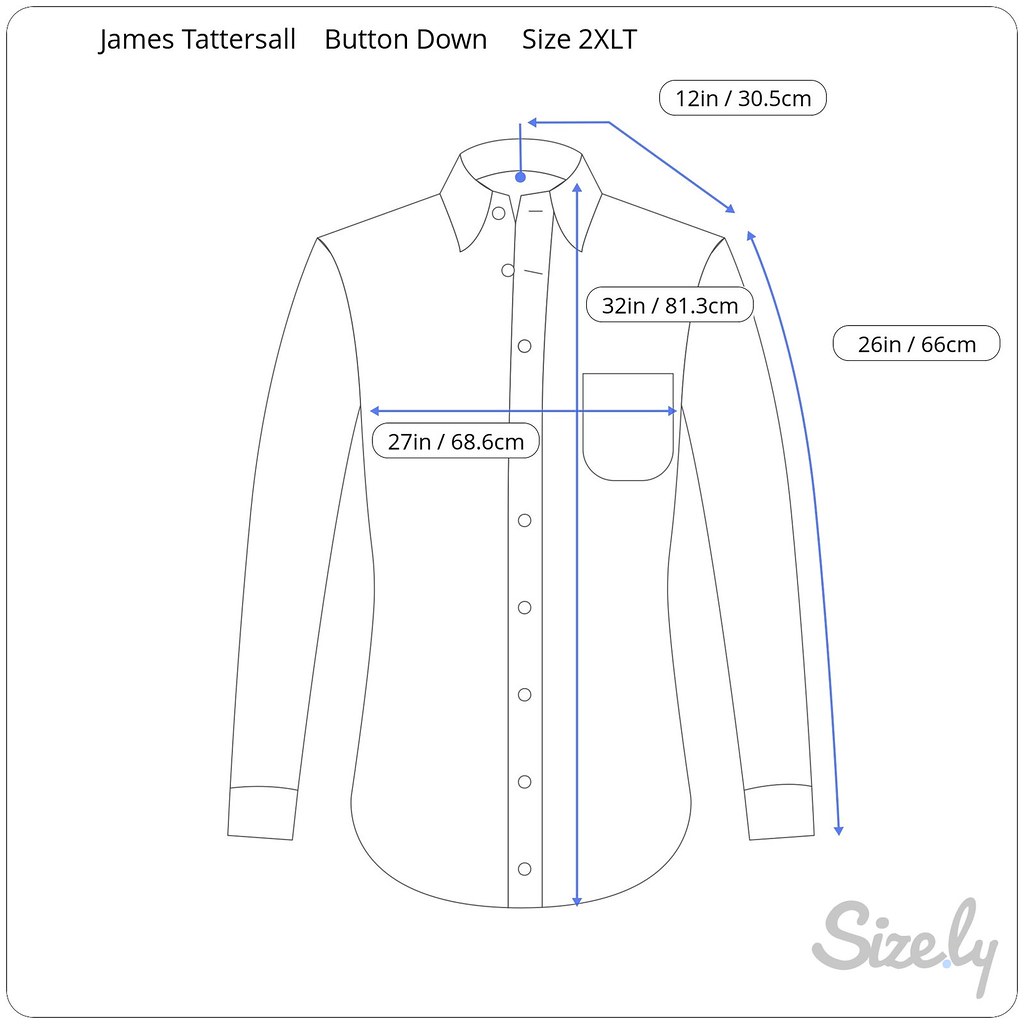The image showcases a detailed diagram of a James Tattersall button-down shirt, size 2XLT, on a white background. Centered in the image is a drawing of a long-sleeve button-up shirt with a collar, button placket, single chest pocket on the left side, and cuffs. The diagram includes various measurements marked by blue arrows and corresponding text bubbles. In the upper left corner, black text reads "James Tattersall, button down, size 2XLT." The measurements detailed are: 12 inches (30.5 centimeters) from the middle of the collar to the shoulder, 32 inches (81.3 centimeters) from the top of the collar to the bottom of the shirt, 27 inches (68.6 centimeters) across the chest area, and 26 inches (66 centimeters) from the shoulder seam to the end of the sleeve. At the bottom of the image, in gray cursive text, is the watermark "Sizely."